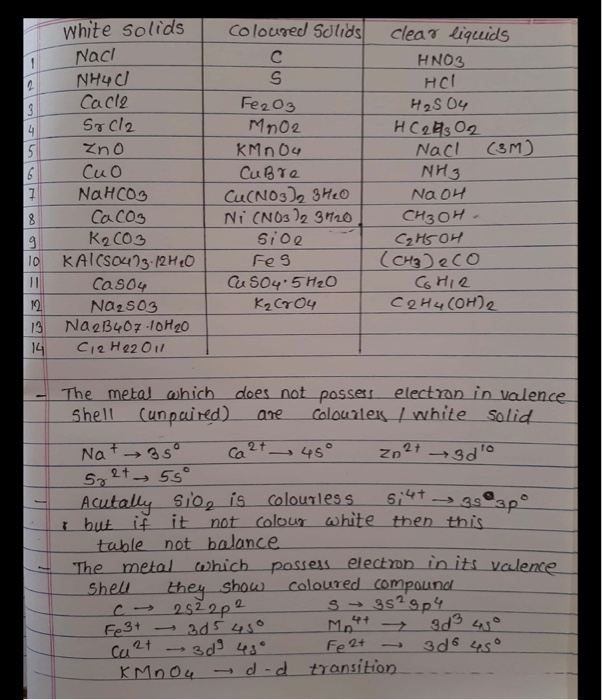This photograph captures a college-ruled notebook page filled with handwritten notes. The page is lined with blue horizontal lines and features red vertical margins on the left. At the top of the page, there is a table organized into three vertical columns labeled "White Solids," "Colored Solids," and "Clear Liquids." Each column contains a list numbered from 1 to 14, detailing various scientific notations corresponding to each category. Examples of these notations include "C" and "Fe2O3." Below this table, additional notes delve into the characteristics of metals based on their electronic configuration. For instance, one detailed note states that metals without unpaired electrons in their valence shell are colorless or white solids, while those with unpaired electrons exhibit colored compounds. Further explanations and scientific notations elaborate on these properties, including specific mentions like "SiO2 is colorless." The detailed handwriting indicates that these are notes likely taken from a textbook or lecture, providing in-depth chemical insights.